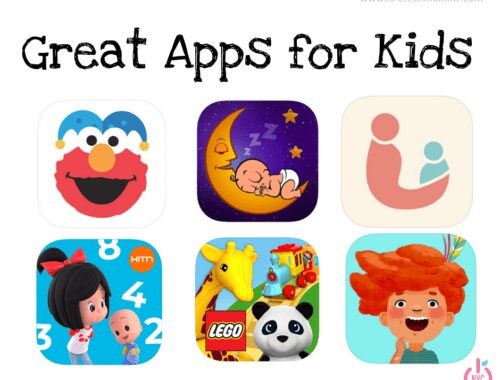This screenshot showcases a banner titled "Great Apps for Kids" in a bold, black font styled to look childlike and handwritten. Below the title, a row of three app icons is displayed. The first icon, set against a white background, features Elmo's face adorned with a blue jester hat, giving a jovial appearance. The second icon, against a purple and black background, depicts a cartoon-like newborn baby peacefully sleeping on a crescent moon, adding a dreamy, nighttime theme. The third icon is a bit more complex, with the lower left corner showing a blue background and cartoon illustrations of a little girl and a baby. To the right of this, the image showcases an app related to Lego. Finally, the last icon presents a red-headed boy against a light blue background, completing the row with a vibrant, playful vibe.